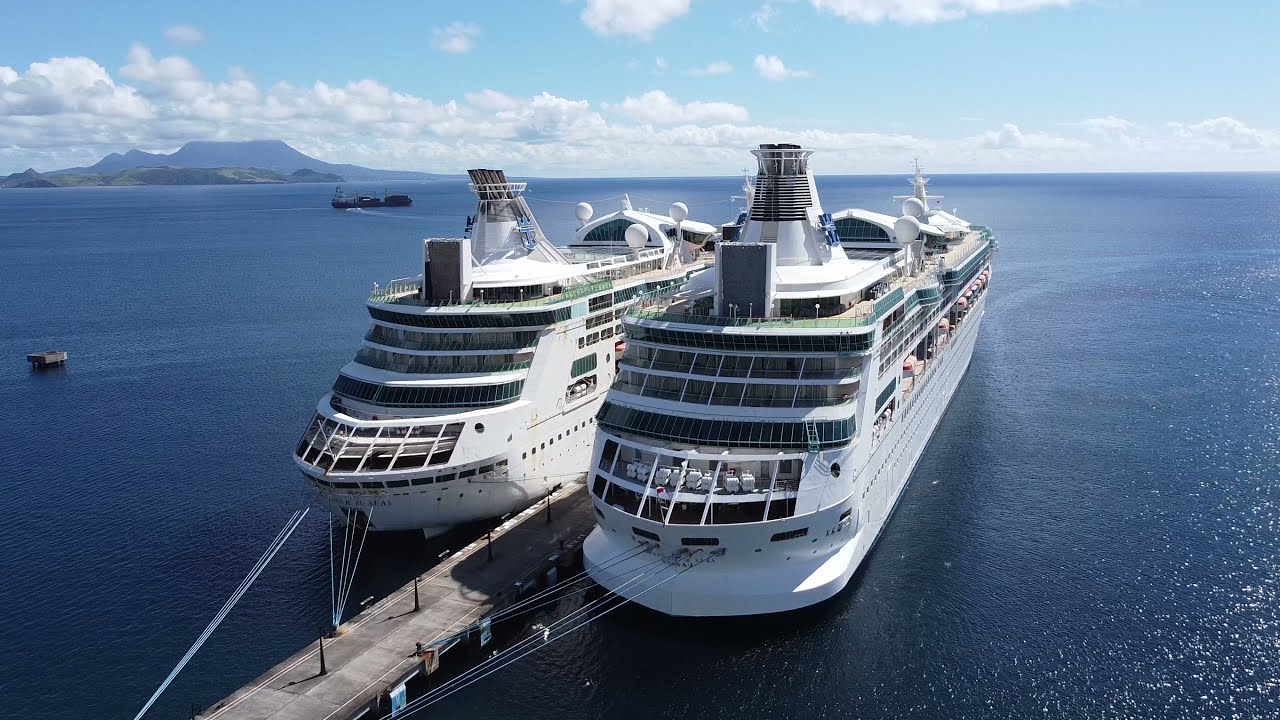This high-definition, color, drone photograph vividly captures two nearly identical, white, multi-level vacation cruise ships docked side by side at a narrow wooden dock. The image is in landscape orientation and depicts a stunning outdoor scene bathed in daylight. The deep blue ocean forms the backdrop of the photo, occupying about two-thirds of the frame. Above this, the light blue sky stretches across the top, dotted with white puffy clouds. To the left, two mountain peaks with greenery at the shoreline are visible on the horizon. Both cruise ships are tethered to the dock with long, white ropes at their fronts. Smaller black vessels can be seen to the left of the cruise ships, adding more detail to the vibrant marina scene. The color palette is a mix of blues, whites, greens, grays, blacks, tans, and yellows, contributing to the photograph's realistic and vivid quality.